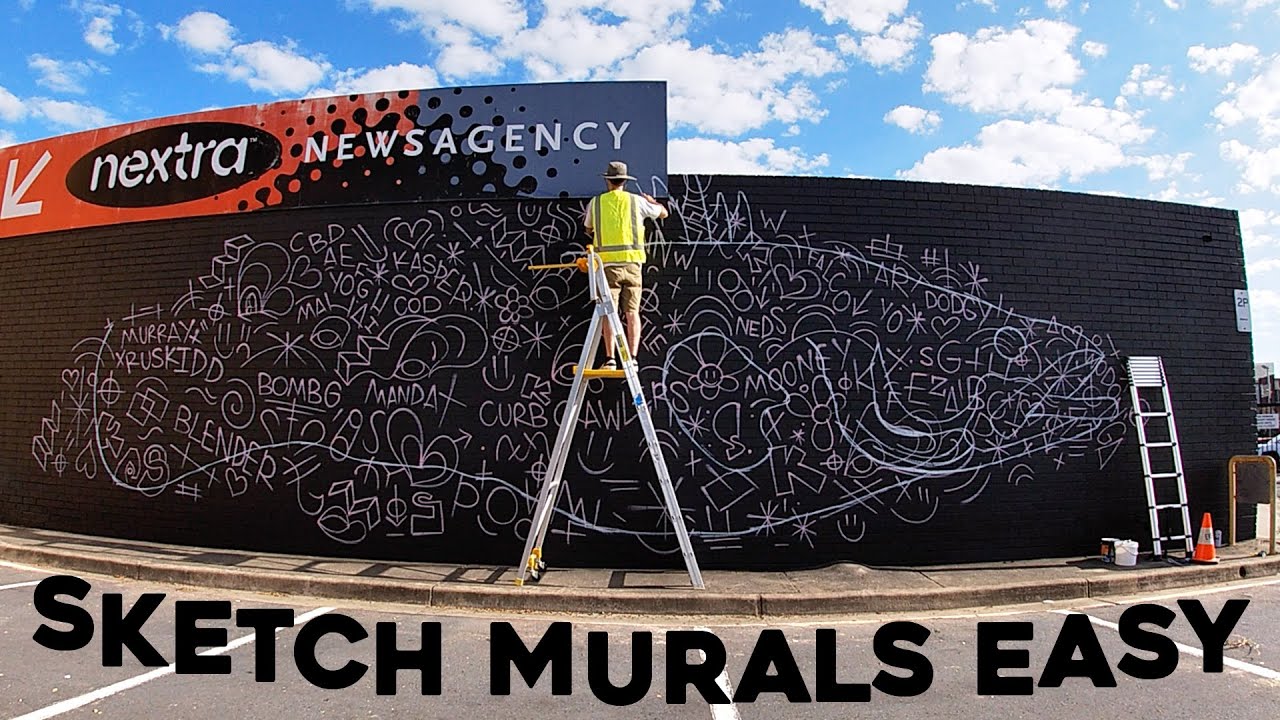In this promotional image, a man in a reflective yellow vest, brown cargo shorts, and a white shirt with a gray-brimmed hat is seen standing on an A-frame ladder. He is carefully sketching intricate white designs, including names like Amanda, Bump, Crab, Moon, and varied shapes like hearts and stars, on the side of a black brick building. The scene is set under a cloudy sky, adding contrasting brightness to the heavily detailed mural. To the right of the muralist, another ladder leans against the building, surrounded by an orange traffic cone and paint buckets. On the top left of the wall, a brightly colored sign for "Nextra News Agency" features a white arrow and bold, eye-catching fonts. Below, large black uppercase letters command attention with the phrase "Sketch Murals Easy." The ground consists of a gray concrete sidewalk and a pavement area, enhancing the gritty urban atmosphere of this street art scene.